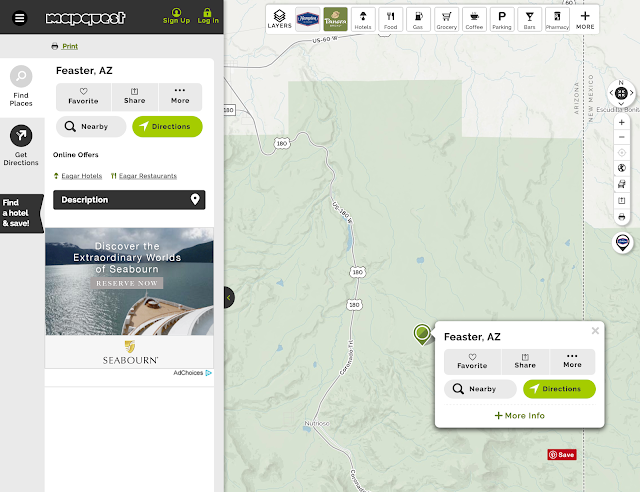This screenshot captures a search for Feaster, Arizona, on the MapQuest website. In the upper left corner, the MapQuest logo is prominently displayed, alongside options to sign up or log in, indicating the user is currently browsing without logging in. Just below, a toolbar features options to print the page, find places, add to favorites, share, explore more, view nearby places, and get directions. An advertisement directly below promotes "Discover the Extraordinary Worlds of Seaborne Reserve," with an "Ad Choices" link prominently displayed.

Occupying roughly two-thirds of the screen, the map highlights Feaster, Arizona, marked clearly as the focal point. A green "Directions" button is available here for easy navigation assistance. At the top of the map, various filters can be toggled on or off, allowing the user to customize the view to show or hide locations for restaurants, rest stops, food, gas stations, grocery stores, coffee shops, and parking areas. Specific examples of these eateries, such as Hampton Inn and Panera Bread, exemplify the types of establishments that can be displayed or hidden according to the user's preferences.